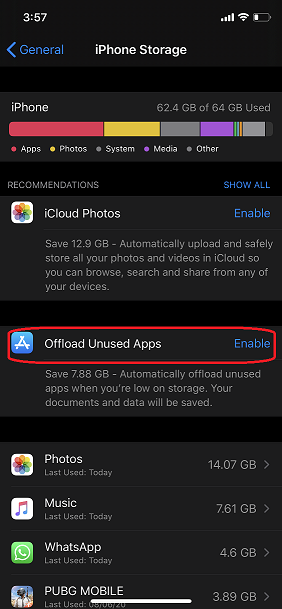In the image, an iPhone is displayed with its settings opened, showcasing the device's storage management screen. The phone is using Dark Mode, resulting in a black background. The storage capacity is nearly full, with 62.4 GB of the 64 GB utilized. The majority of this space is occupied by apps, photos, and the system itself. Specifically, photos are taking up a significant 14 GB, while music accounts for 7.5 GB. 

Media is separately classified but also occupies a considerable amount of space. To address this issue, options to optimize storage are highlighted. The option to enable iCloud Photos is shown, which promises to free up 12.9 GB by automatically uploading and offloading photos from the device. Another option, "Offload Unused Apps," indicates it can save 7.8 GB by removing seldom-used applications. It's evident that the user must take action, such as transferring photos or enabling these storage-saving features, to prevent the phone from running out of space and potentially affecting performance.